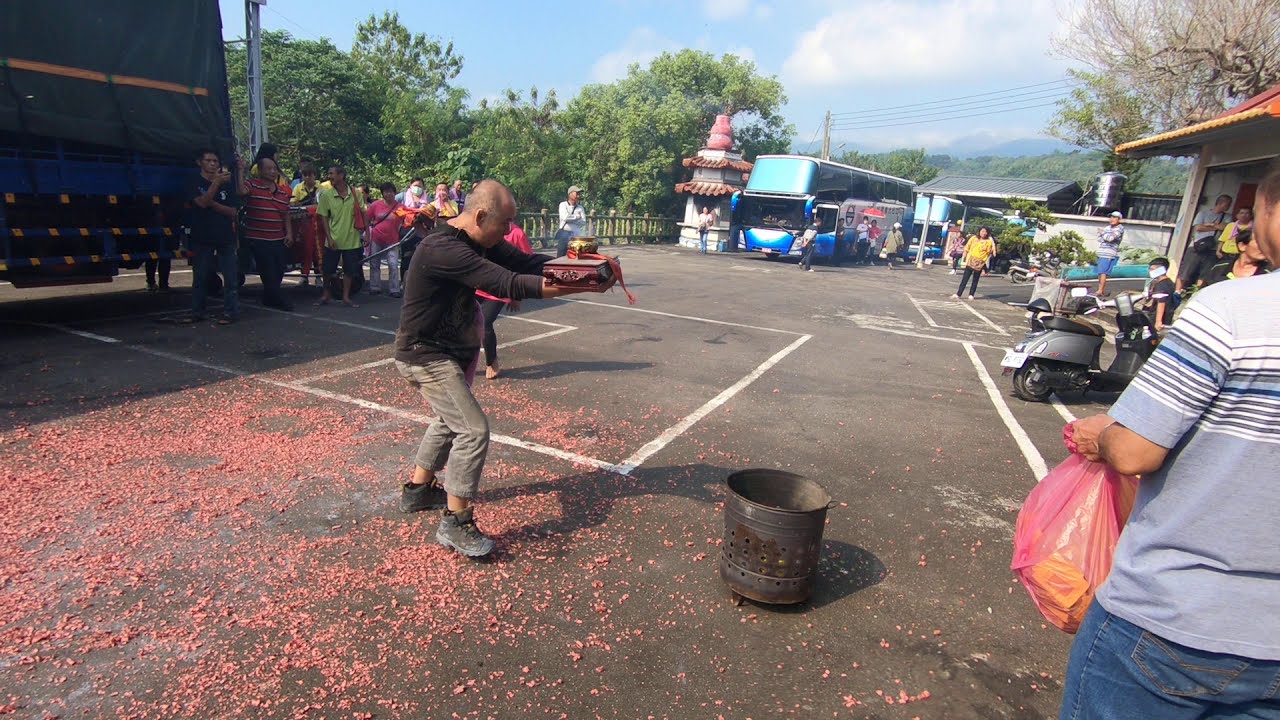In an outdoor scene set in what appears to be an Asian country, a man dressed in a black long-sleeved shirt, gray jeans, and work boots stands at the center of attention. He holds a decorative, traditional-looking box, with a gold object resting on a red cushion atop the box, extending his arms towards a rusty metal bin that seems intended for burning items. Surrounding him in what resembles a parking lot are spectators, including a person in a gray and white striped shirt clutching a reddish bag, likely capturing the event on video. The ground around the man is strewn with red debris, possibly smashed petals or berries. In the background, a blue bus, some trees, and Asian-style buildings add context to the setting, suggesting a small festival or ritualistic gathering.